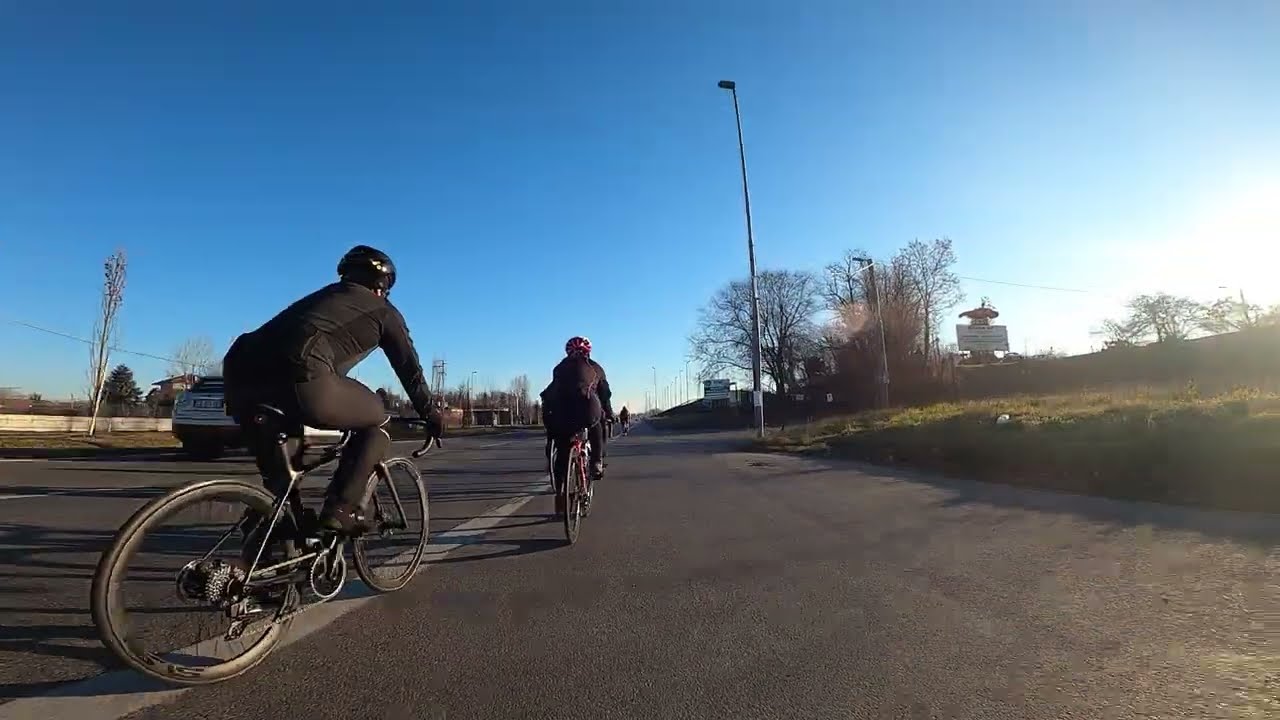In this image taken during the day, we see a clear blue sky without a cloud in sight, indicating bright and sunny conditions. The scene depicts a road with a white line running from the lower left corner toward the center, guiding our view to two cyclists riding closely together. Both cyclists are dressed in all-black outfits, including long-sleeve shirts, long pants, and black helmets. The first cyclist is on a black bike, while the second one is on what appears to be a bike with some red detailing, possibly a red helmet or bike parts, making it somewhat distinguishable despite the distance.

To the left of the cyclists, there's a partially visible white car, suggesting it's either parked or passing by, and alongside it, several trees can be seen. These trees are a mix of deciduous ones without leaves, hinting at a fall or early spring season, and an evergreen tree further in the background. The right side of the road includes patches of grass, more leafless trees, and a tall streetlight towering above the scene. Additionally, a sign is visible on the right, although its details are indistinguishable. In the distant background, other indistinct figures and possibly other cyclists can be seen, adding depth to the image.